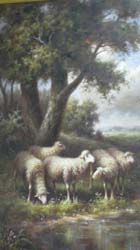This is a very small, blurry illustration, possibly a cropped and resized painting, depicting an outdoor scene with muted pastel colors including green, blue, cream, yellowish cream, brown, and gray. In the center of the image, five white, woolly sheep stand in various positions, with one grazing. These sheep are positioned against a shoreline at the bottom right, where water, possibly a lake or pond, reflects their faint, shadowy figures. The expansive background features a large, leafy tree, possibly an oak, on the left side, accompanied by various shrubs and vegetation. Overhead, a light blue sky is dotted with puffy clouds, adding to the serene, pastoral atmosphere.